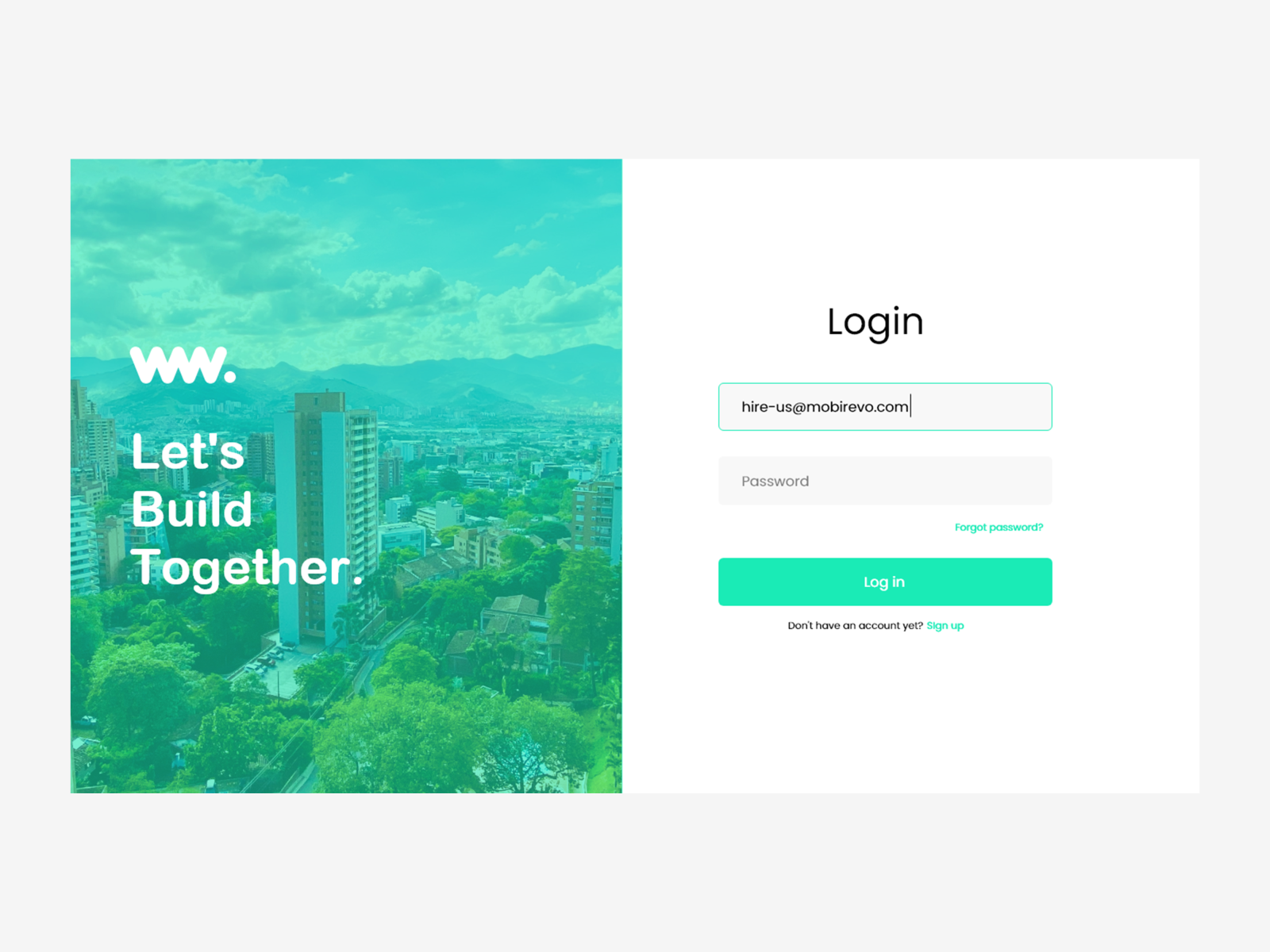A screenshot portrays a vibrant login page for a platform called "WW: Let's Build Together." The background of the login area is painted in a serene blue hue featuring an illustrated cityscape. Tall buildings are surrounded by lush green trees, with majestic mountains and fluffy clouds gracing the distant skyline. 

To the right of this welcoming scene, the login form is prominently displayed on a crisp white background, framed by a subtle gray outer background. The form elements include fields for "Username" and "Password," along with links for "Forgot Password" and "Sign Up" options, catering to both returning and new users. The word "Login" is highlighted in bold black letters, ensuring it catches the user's attention immediately. The platform encourages teamwork and creativity, as emphasized by the inviting tagline "Let's Build Together."